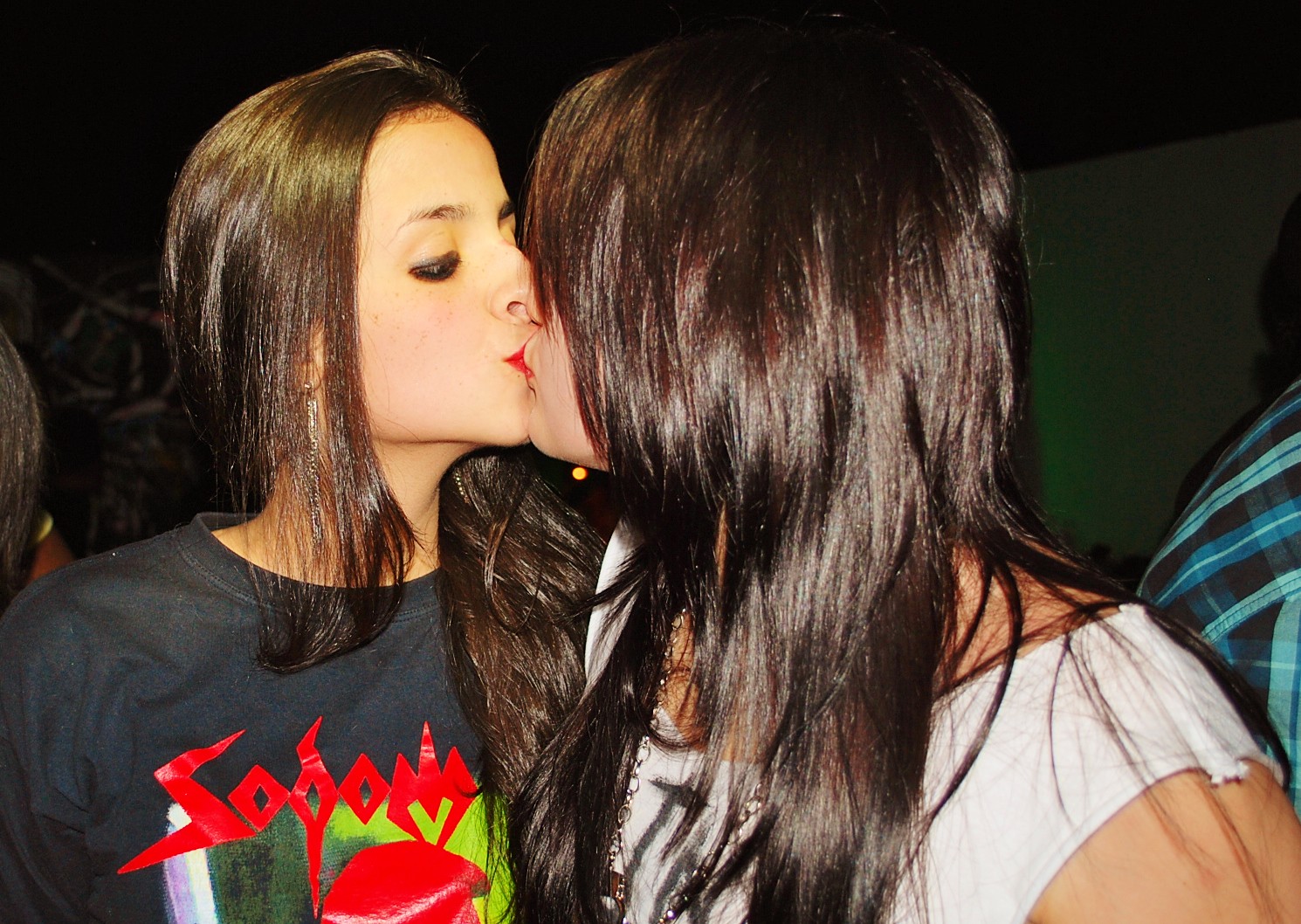In this photograph, two women are sharing a kiss in what appears to be a dark room, perhaps at a party, surrounded by indistinct figures and shadows in the background. The woman on the left, with light-colored skin, is clearly visible. She has shoulder-length, shiny brown hair, dark eyeliner, and bright red lips. She wears a black scoop neck t-shirt featuring the word "SODOM" in bright red letters, along with a design that includes additional red, green, white, and darker colors. She also has long silver earrings. The woman on the right, whose face is partially obscured but shows light-colored skin and a slender build, also has long, straight, shiny brown hair. She is dressed in a white sleeveless t-shirt and wears multiple necklaces. The crowd behind them is difficult to make out, with only glimpses of clothing like a blue plaid shirt adding to the ambient setting.